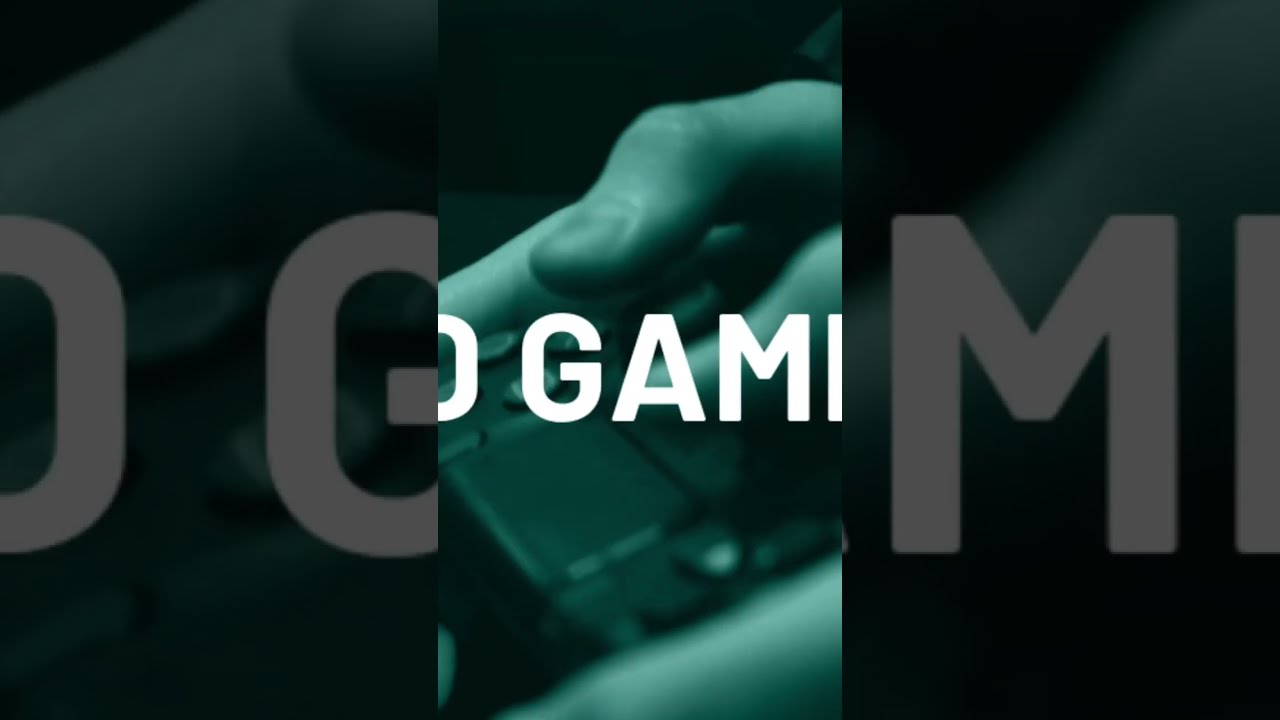This image is a close-up, grayscale still featuring hands, likely white-skinned, gripping a black video game controller, possibly an Xbox controller. The central section of the image, tinted green, shows the hand illuminated as though a green light is shining on it. Across the hand, white, all-capital sans-serif text is partially overlaid, displaying the letters O, G, A, M, and I. The left and right segments of the image are zoomed-in and darkened sections of the main picture, with the left side showing the letters M and I, and the right side showing O and G. The setup suggests that the image is a screenshot from a video where the text ‘video gaming’ is being panned across the screen, captured mid-transition.